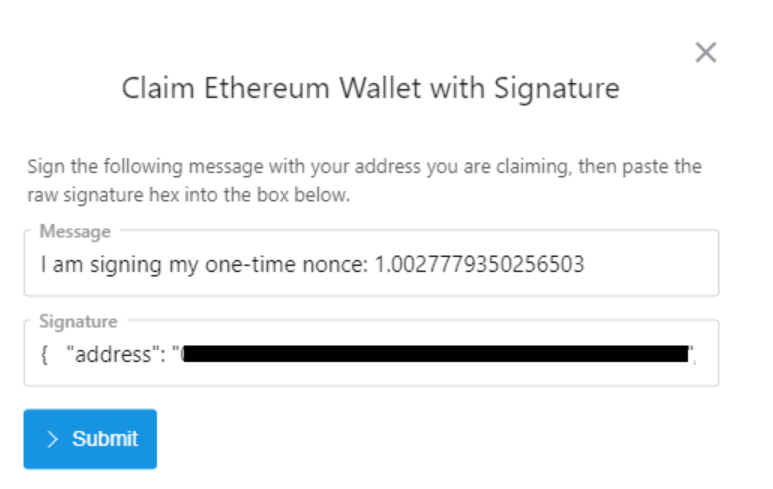The image appears to be a partial screenshot, possibly taken from a mobile device. In the top right corner, there's a gray 'X' icon likely intended to close this section of the app. Below this, there is a header labeled "Claim Ethereum Wallet with Signature." 

The instructions provided beneath this header are as follows: 
"Sign the following message with the address you are claiming, then paste the raw signature hex into the box below." 

The message for the signature reads:
"I am signing my one-time, once, NONCE: 1," followed by a series of numbers.

Below the message box, there is a section for the "Signature." It starts with an opening brace and includes the lowercase word "address" followed by a colon and quotations. The address itself seems to have been redacted with a black rectangle hiding the text, enclosed in double quotes, followed by a comma.

At the bottom of the screenshot, there is a medium blue button with a white right arrow and the word "Confirm" in white.

This appears to be a prompt for verifying and claiming an Ethereum wallet through digital signature verification, where some sensitive information has been intentionally obscured.